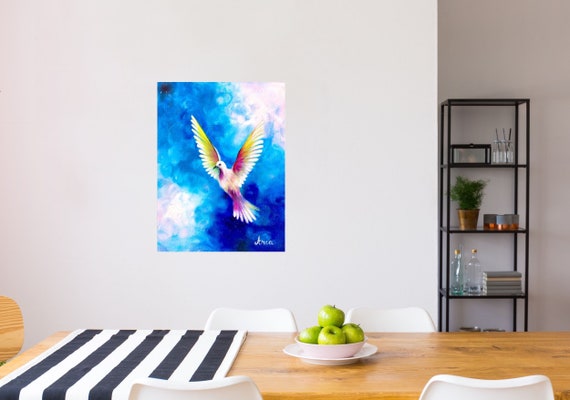The photograph depicts a serene dining room scene with a light wooden rectangular table occupying the bottom fourth of the image, stretching from left to right. Draped over the left side of the table is a vertically striped cloth in dark blue and white. At the center of the table sits a white plate holding a white bowl filled with approximately five green Granny Smith apples. Surrounding the table are four white chairs with resin backs, two at the front and two at the back.

Dominating the background, the back wall takes up the top three-fourths of the image and is painted white. Slightly to the left of the center on this wall hangs a vibrant watercolor painting of a dove in flight. The dove is adorned with intricate details, including red, yellow, and purple trimming on its feathers, set against a backdrop of bright blue, royal blue, dark blue, and turquoise hues, with some white clouds.

On the right side of the image, there is a recessed area featuring a simple metal shelving unit with three tiers. These shelves hold a variety of items including plants, vases, books, flowers, and glass bottles, adding a touch of eclectic charm to the room. The overall ambiance suggests a thoughtfully decorated dining area within someone's home.